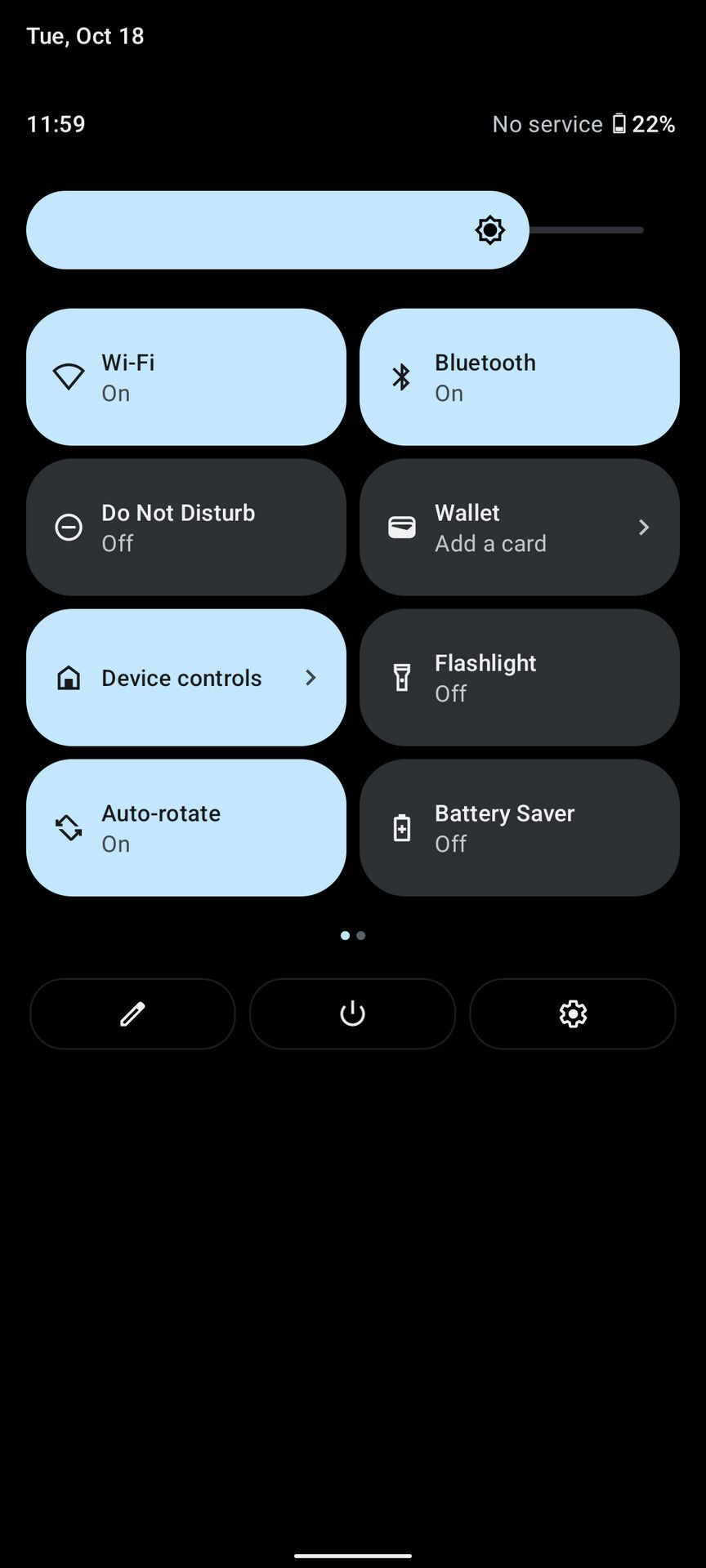The photograph is a screenshot taken from a smartphone, predominantly featuring a black background. The display indicates "TEU," signifying Tuesday, October 18th, with the time shown as 11:59. In the top-right corner, the phone status shows "No Service" and a battery level of 22%. 

Central to the image, there's a periwinkle-colored input field accompanied by a gear icon, suggesting access to settings or further options. Below this, the screen is divided into a grid with two columns of four rounded rectangles, resembling clickable buttons.

In the top left of this grid, the Wi-Fi is turned on, followed by Bluetooth turned on in the top right. The next item in the left column is a dark grey/black box indicating "Do Not Disturb" is off, paired with "Add a Card" under Wallet on the right. 

Continuing down, the next row on the left reveals "Device Controls" in periwinkle, and "Flashlight Off" in black. The final row displays "Auto Rotate" in periwinkle, indicating it is on, and "Battery Saver" in black, showing it is off.